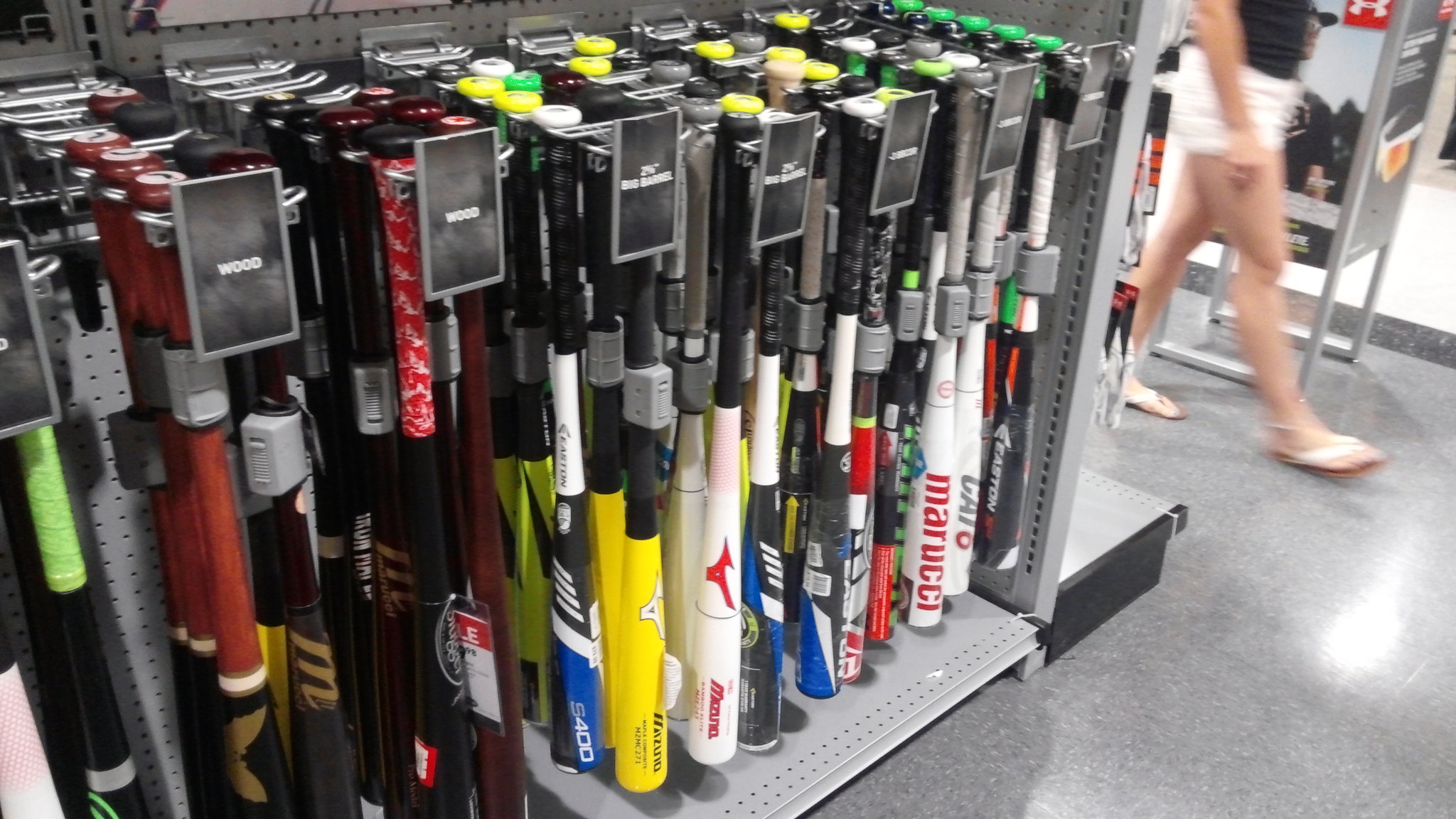The image depicts a landscape-oriented photograph taken inside a sporting goods store, showcasing a large display of baseball bats. The bats are organized on a gray metal shelving unit with pegboard backing and are arranged in several rows, each row clearly labeled with small black signs featuring white letters that identify the bat material—wood or aluminum. Various models, including notably named ones like Marucci and S400, are visible, and the bats come in multiple colors such as white, black, blue, and yellow. They are suspended by their handles, pointing downward from hooks.

In one section of the image, a woman dressed in white shorts, white sandals, and a black tank top is seen walking down an aisle. Her upper body is not fully visible, adding a sense of motion blur to the picture. The store's flooring is a dark gray linoleum. Adjacent to the bat rack, there is a display of batting gloves, and a large advertising sign with images stands in the aisle next to her. The photo provides a comprehensive view of the variety and arrangement of bats available for shoppers to select from.